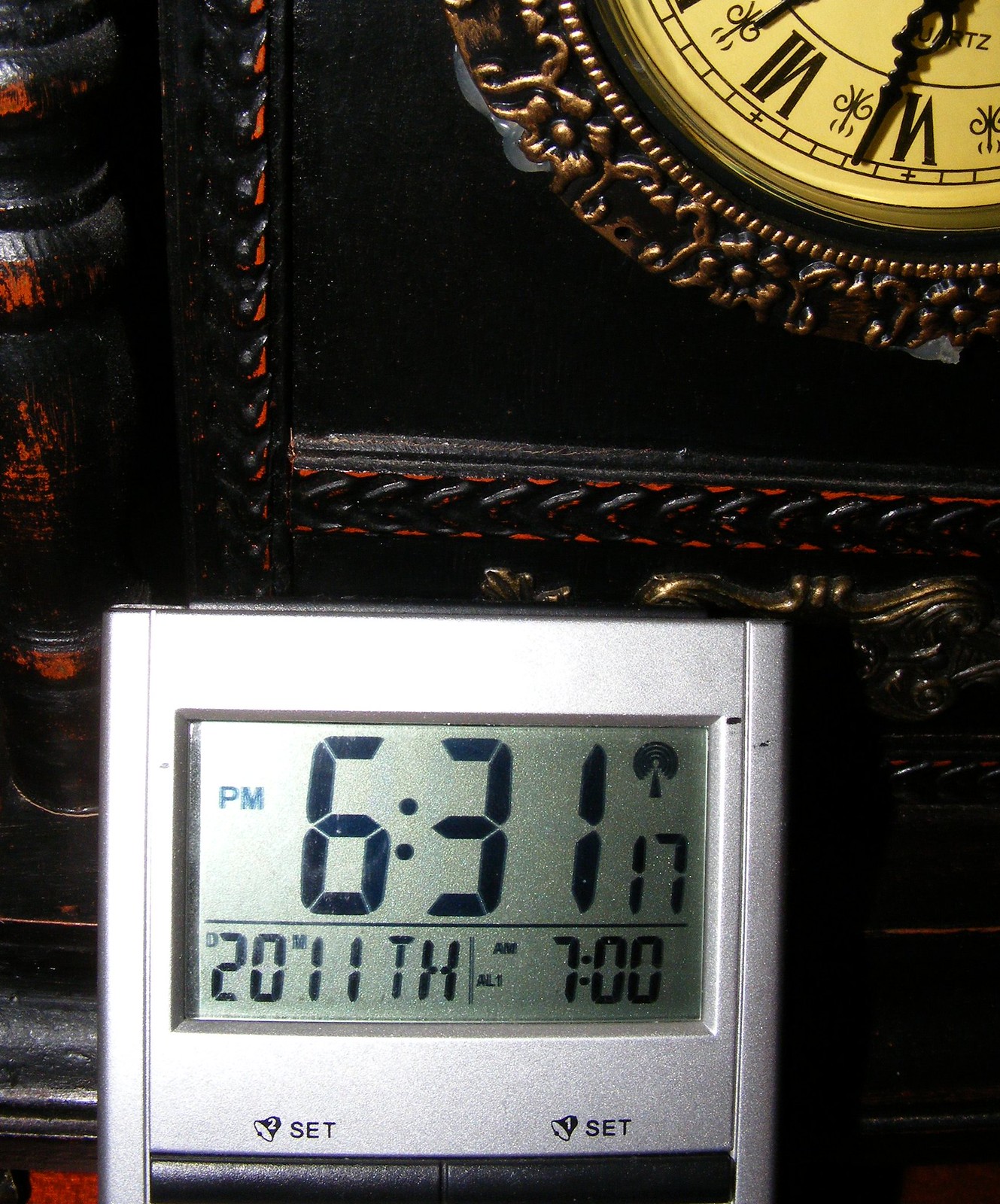This photograph captures two distinctive clocks. In the foreground, occupying the lower half of the image, is a digital clock encased in silver plastic. The digital display prominently shows the time as 6:31 PM. Below it, smaller lines and text detail the day (Thursday), date (20th), month (November), and indicate that an alarm is set for 7:00 AM. The digital clock also features two black buttons labeled "Set 1" and "Set 2" for alarms. In the background, partially obscured, is the lower left quadrant of an ornate analog clock. This clock has a dark, possibly wooden case with red highlights and brass hardware, while its face is pale yellow. The visible Roman numerals VII (7) and VIII (8) are marked in black, with elegant black hands completing its sophisticated appearance.